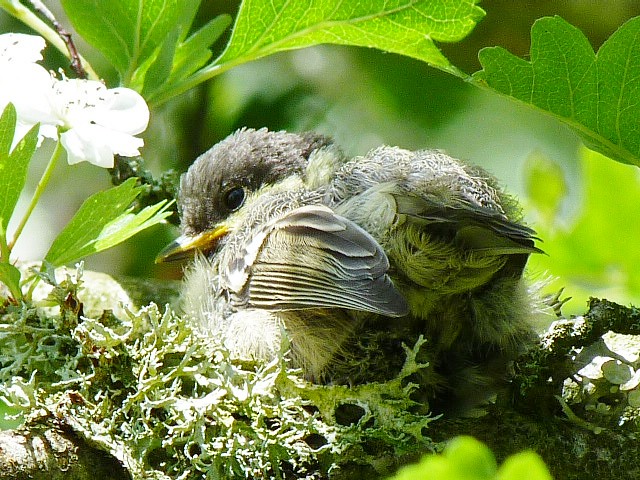The photograph captures a serene outdoor scene in the middle of the day, primarily focused on a fluffy baby bird with fluffed-out feathers. The bird, positioned directly at the center of the image and facing slightly left, showcases colors such as black, gray, yellow, and a touch of white. We can distinctly see its dark, expressive eye and a black and yellow beak. The bird is perched comfortably on green tree leaves, with its tail facing us. Sunlight filters down gently onto its face, adding a soft radiance. Surrounding the bird, there is an abundance of lush greenery, including various types of bushes, plants, and a couple of white flowers visible to the left. The background is blurred to emphasize the detailed and vividly clear foreground, drawing focus to the bird and the immediate foliage around it.